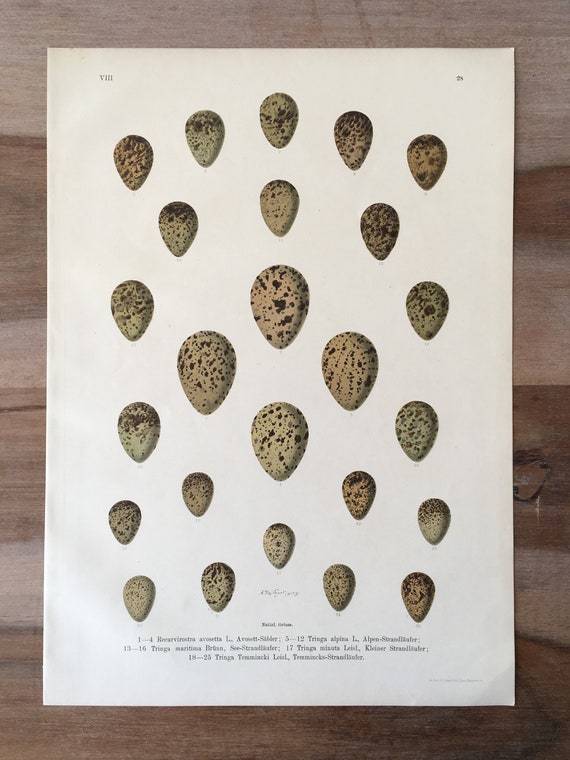The image depicts a detailed print art showcasing bird eggs, specifically sandpiper eggs, arranged in a structured geometric pattern. The eggs are oval-shaped, resembling guitar picks with the narrower ends pointing downward. They are colored in a beige tone with brown spots, and the larger eggs are centrally positioned while the smaller ones form a surrounding perimeter. The eggs are placed on white paper, itself set against a grayish-brown hard surface, which resembles stone or granite with black splotches. At the bottom of the image, there's text in small, barely readable font that appears to be a classification key, listing numbers 1 through 25 with specific labels such as "Tringa Alfina." Each egg correlates to these numbers, providing an organized method for identification, emphasizing the ornithological style of the artwork.